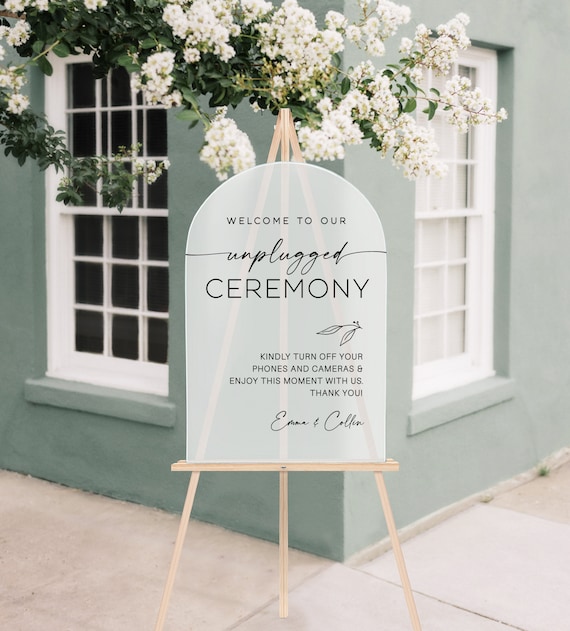This detailed image captures a serene outdoor scene in front of a light gray building, positioned so the corner faces the camera, revealing two walls with white windows. The left window shows a dark interior, while the right window has a white background. Above the building, a lush green tree adorned with white flowers extends across the top of the picture. Dominating the foreground is a wooden tripod stand, extending from the bottom almost to the tree's canopy. At its midpoint, there's a wooden crossbar with a headstone-shaped sign. The sign reads, "Welcome to our unplugged ceremony. Kindly turn off your phones and cameras. Enjoy this moment with us." On the ground, which features large tan tiles, the setting radiates tranquility, suggesting it might be a venue for a special ceremony, possibly a wedding or small church event.